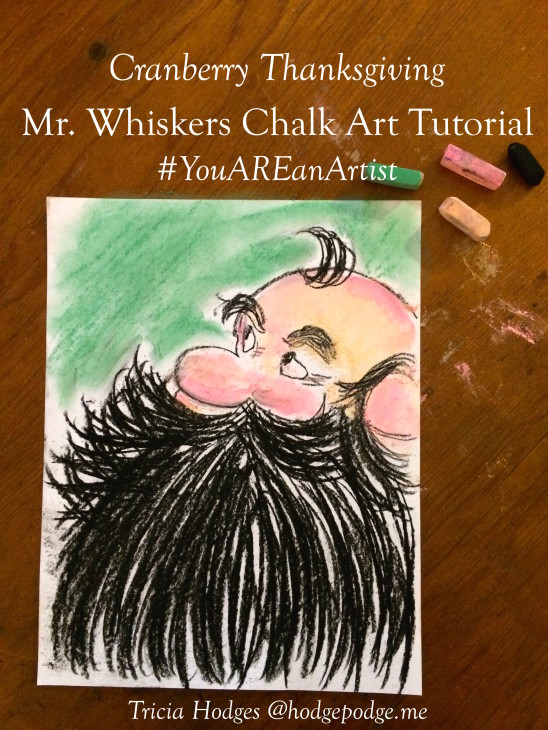The image features a chalk drawing titled "Cranberry Thanksgiving" at the top, followed by the text "Mr. Whiskers Chalk Art Tutorial" and the hashtag "#youareanartist." The drawing depicts a mostly bald man with a single tuft of black hair atop his head, bushy black eyebrows, a bulbous nose, and an enormous, wispy black beard that obscures much of his face. The artwork has a green chalk background. To the right of the drawing are four pieces of used chalk in green, pink, yellow or orange, and black, indicating the pastels used in the artwork. These elements rest on a medium-toned wooden table, possibly cherry wood. At the bottom of the image, the artist is credited as Tricia Hodges with the handle "hodgepodge.me."